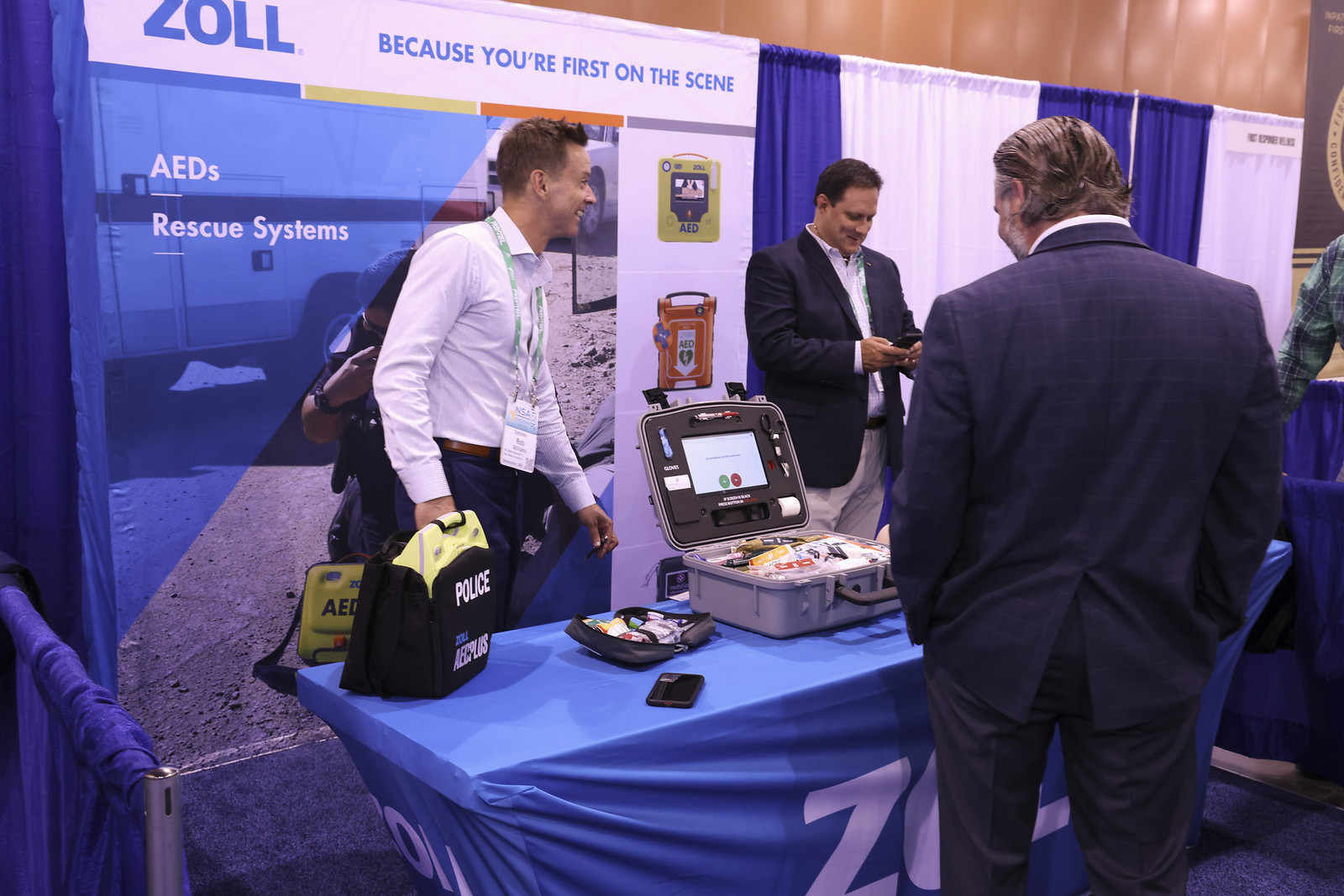In this rectangular, landscape photograph from a convention or trade show, three men are gathered around a display booth for the company Zoll, which specializes in AED rescue systems. Emphasizing safety and emergency response, the display prominently features the slogan, "Because you're the first on the scene," alongside the company's logo, "ZOLL," in blue.

The booth is set with a medium blue tablecloth, behind which two men stand. The man to the left wears a white collared shirt with blue pants and a lanyard, his sleeves rolled down to his wrists, and he is smiling while looking to his left. The man in the middle of the image wears a blue sports coat and tan pants and is engrossed in his cell phone. Both exhibit a business casual appearance devoid of ties.

On the table, there is a black bag with the word "POLICE" printed in white font and an open briefcase containing emergency devices, including a digital screen and various accessories. In front of the table, facing away from the camera, is another man in a suit with his hands in his pockets, attentively studying the digital screen within the briefcase.

The scene is framed by blue and white curtains and cushioned brown walls, underlining the professional and formal environment of the trade event where innovative emergency solutions are being presented and presumably pitched to potential investors or interested parties.